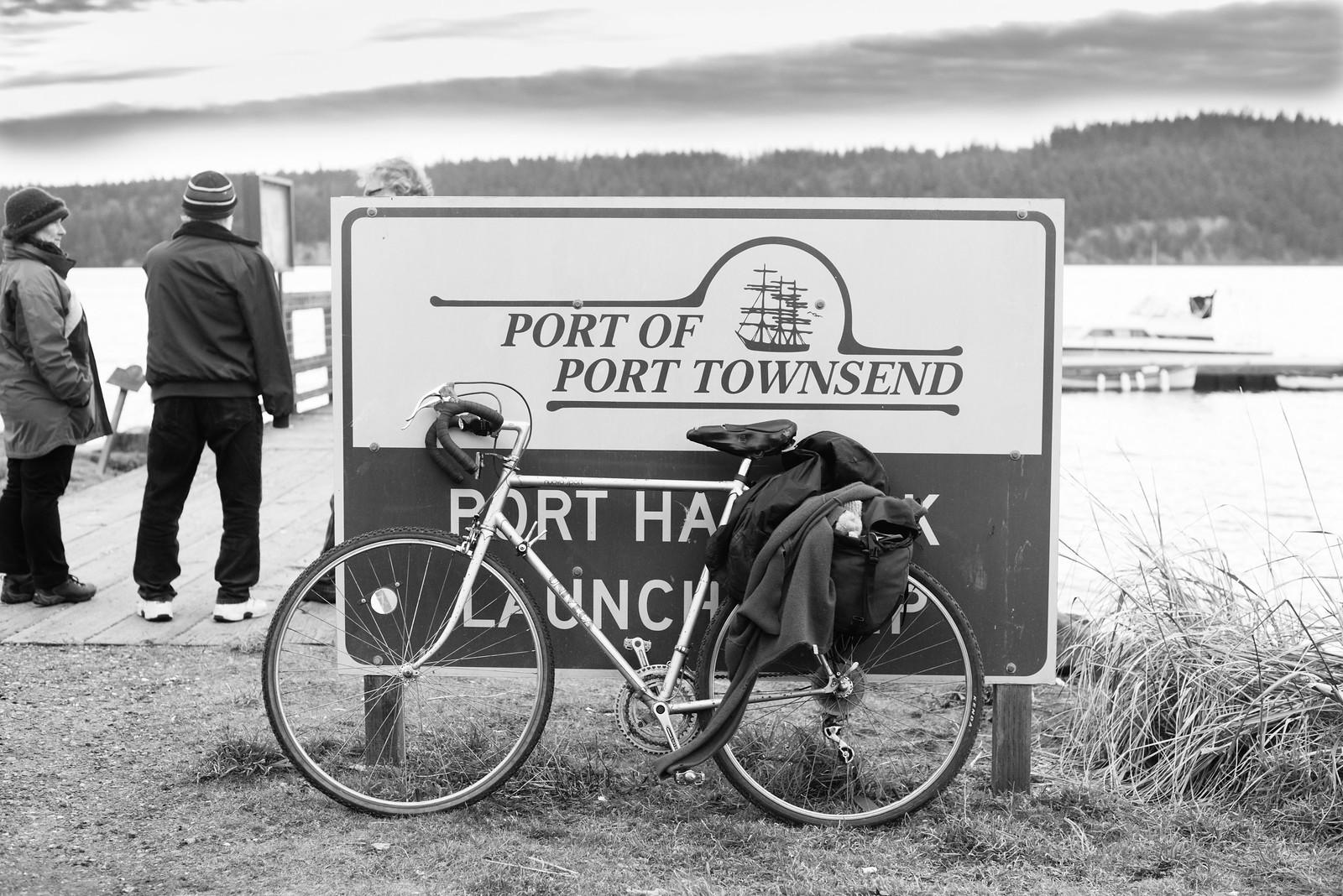The black and white photograph prominently features a sign at its center, held upright by two wooden stakes on either side. The sign, rectangular in shape, reads "Port of Port Townsend" against a presumably white background, although the black and white nature of the image makes it difficult to be certain. At the top of the sign, above the word "Townsend," is a silhouette of an old-fashioned ship, reminiscent of Viking-era vessels, with a few wrapped sails. Directly in front of the sign is a silver bicycle, partially obstructing some of the text at the bottom of the sign, which also includes the words "launch" and "something."

The bicycle has a jacket and a backpack draped over its rear wheel. To the left of the sign stands a couple dressed in warm clothing, including hats, coats, scarves, and beanies, suggesting the photograph was taken in winter or late fall. The couple is facing away from the camera, with one person partially obscured by the sign except for their head. In the background, there is a visible deck extending out to a body of water, possibly a lake or river, with another boat docked nearby on the right side. The water appears white in the photograph, blending seamlessly with the docked boat. Beyond the water, a hill or small mountain range covered in trees stretches across the horizon, with a sky filled with various shades of gray clouds. The area in front of the sign is grassy, adding to the scene's natural setting.